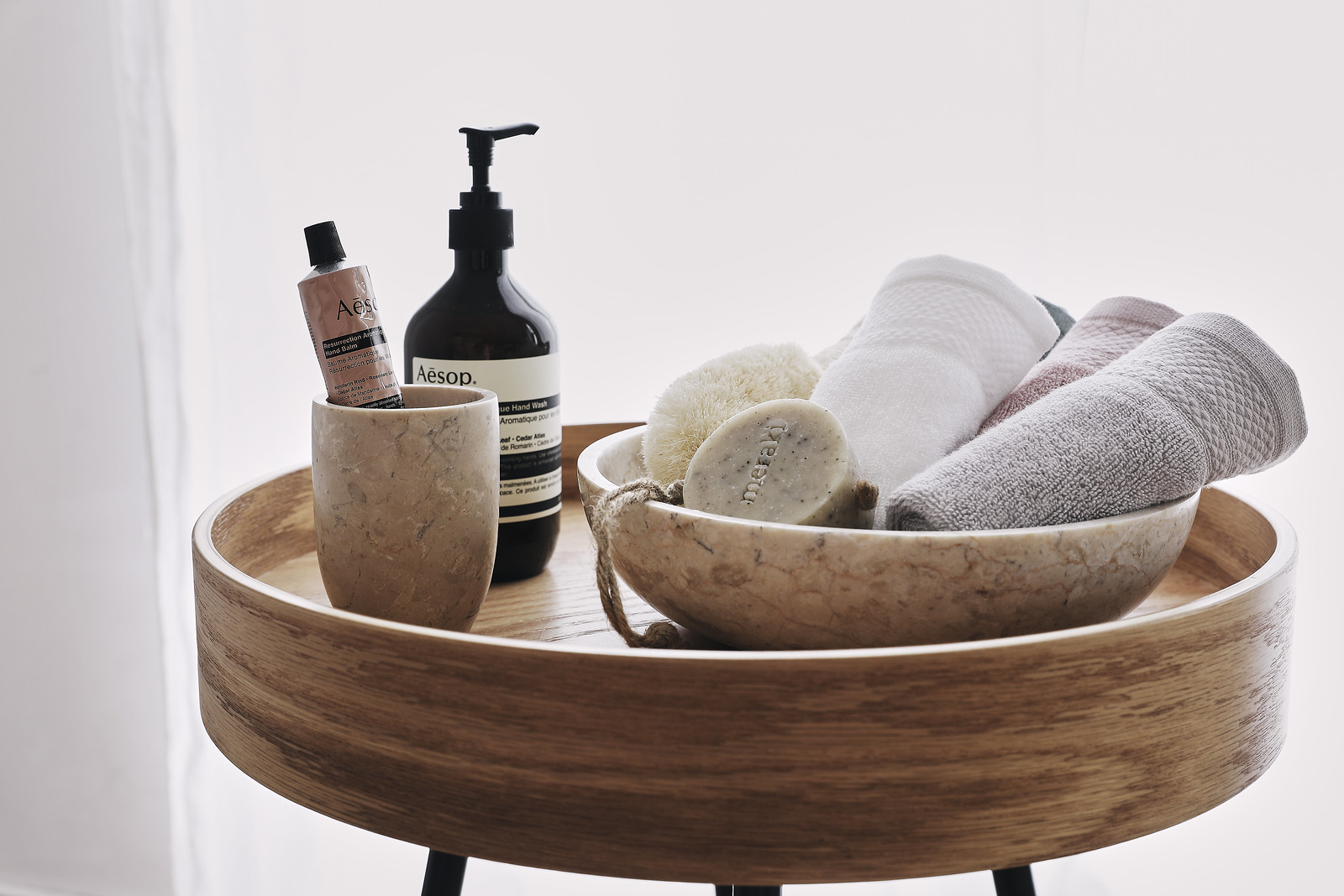The image showcases a serene spa day setup with a crisp, white background that is accentuated by soft shadows, hinting at the presence of a nearby wall in a darker gray shade. Central to the scene is a wide, round table featuring a stunning marble bowl filled with neatly rolled towels in white, gray, and a delicate light pink. Adding to the luxurious vibe is a circular soap labeled "Meraki" and a beige-tan loofah with a subtle tag. Complementing these items is a stylish marble mug with a captivating texture of brown, tan, beige, and coral hues, which holds a tube of Aesop product. Positioned behind the mug, nestled between the marble bowl and the mug, is a sleek black pump bottle of hand wash, adorned with a white label with extensive black text, and a distinctive section of white font on a black background.